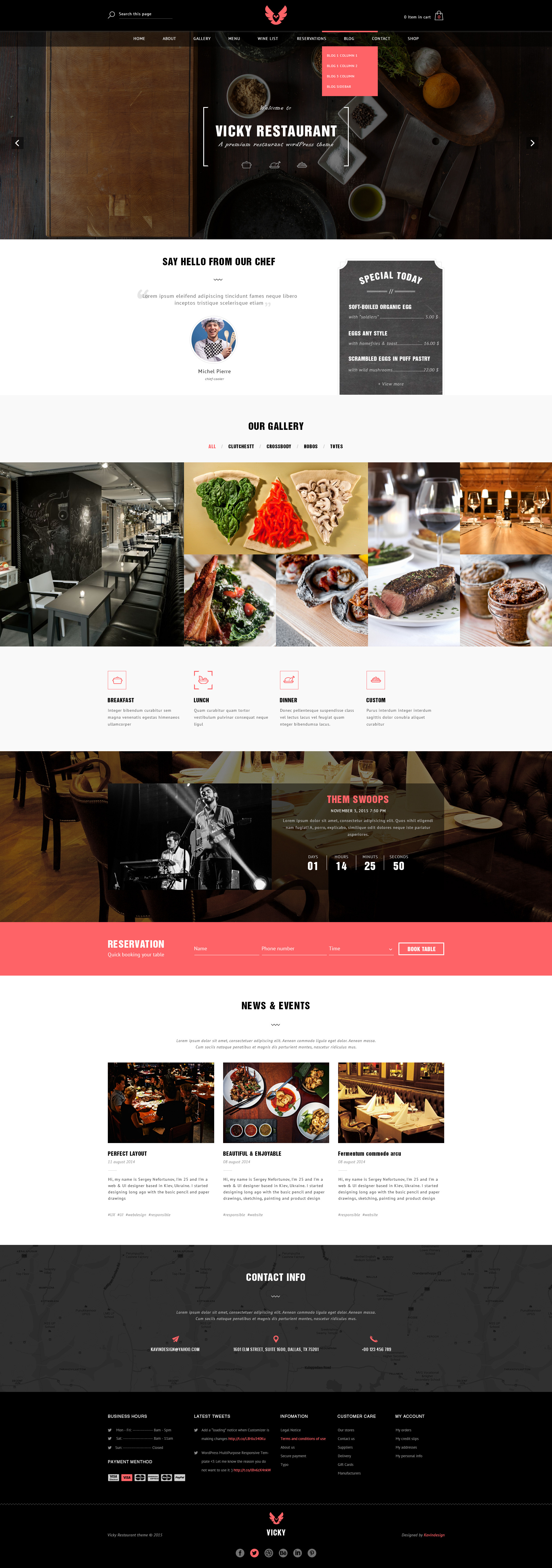This is a detailed screenshot of a restaurant's website. At the top, a black bar spans the entire width of the page, centrally featuring a prominently red logo. Below this bar, there is a semi-transparent black navigation menu that includes nine white text buttons for easy access to different sections of the website. 

Directly beneath the navigation bar, an image slider showcases an appealing table setting with plates and cutlery, enticing visitors with a glimpse of the dining experience. This banner prominently displays the text "Viki Restaurant" framed by decorative brackets on either side. 

The section below the image slider is divided into two distinct segments: On the left, a white section warmly invites visitors with the message "Say Hello From Our Chef." On the right, a complementary grey box titled "Special Today" lists three enticing menu items in striking white text, piquing interest and appetite.